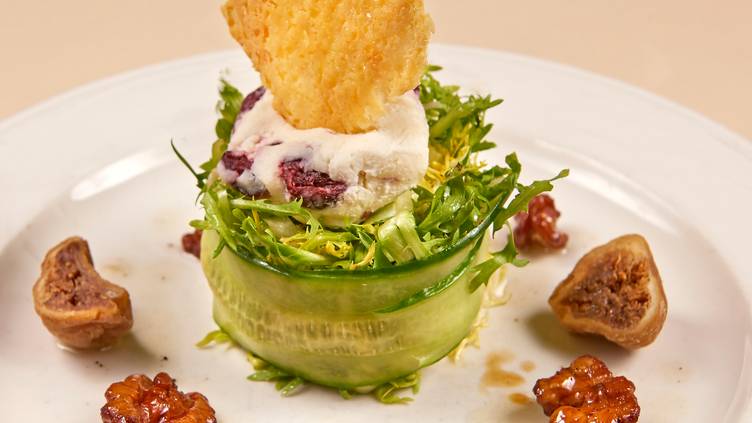The image features a white ceramic plate positioned on a beige table. At the center of the plate is an intricately presented dish comprising various elements. The focal point appears to be a small pouch-like creation, enveloped in green leaves, possibly thinly sliced zucchinis, which may contain shredded vegetables. This central object is topped with a potato chip and a white, raspberry-colored cream or bread. Surrounding the main item are what appear to be scattered candied walnuts and small chunks of bacon, providing hints of red and brown. The overall color palette of the dish includes vibrant greens, whites, tans, and touches of red and brown, giving it an elegant and possibly gourmet feel.